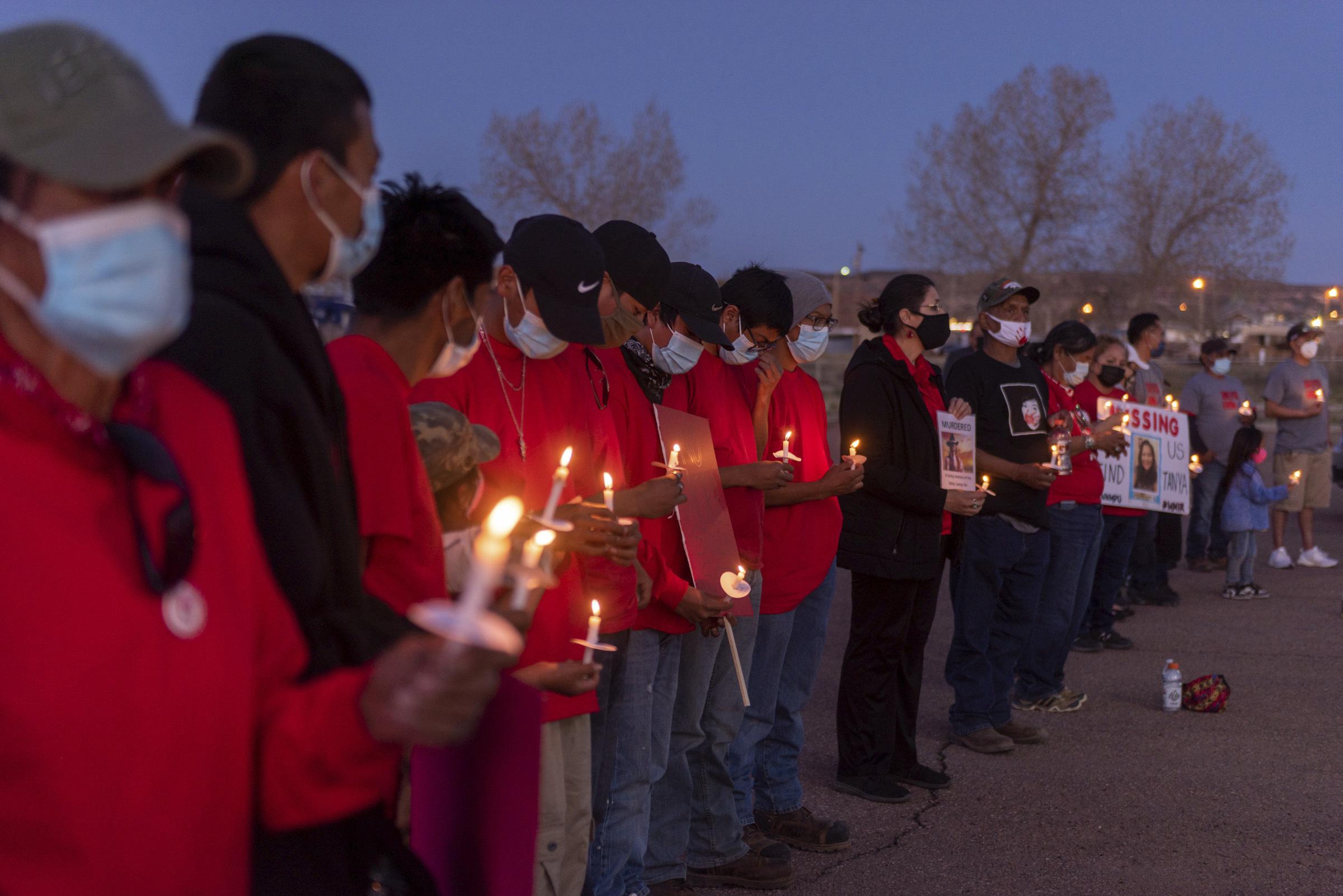In this powerful and emotional image, approximately 30 individuals, comprising both men and women, are gathered outdoors at sunset for a candlelit vigil. Each person is solemnly holding a candle, their expressions marked by sadness and concern. They wear face masks, suggesting this occurred during the COVID-19 pandemic, and are dressed predominantly in red, black, and gray attire. The group appears to be of Filipino or Asian descent, with some people potentially in traditional clothing. At the far right end of the line, a woman displays a large "MISSING" poster featuring a photograph of a young girl, presumably named Lisa. She stands amidst bare trees under a transitioning sky from daylight to dusk, reinforcing the somber atmosphere. Among the group, a child also holds a candle, underscoring the poignancy of the scene as they all hope to bring the missing girl back home. The presence of items like a spray can and a helmet on the ground adds to the realism, highlighting the community's earnest efforts in their search and vigil.